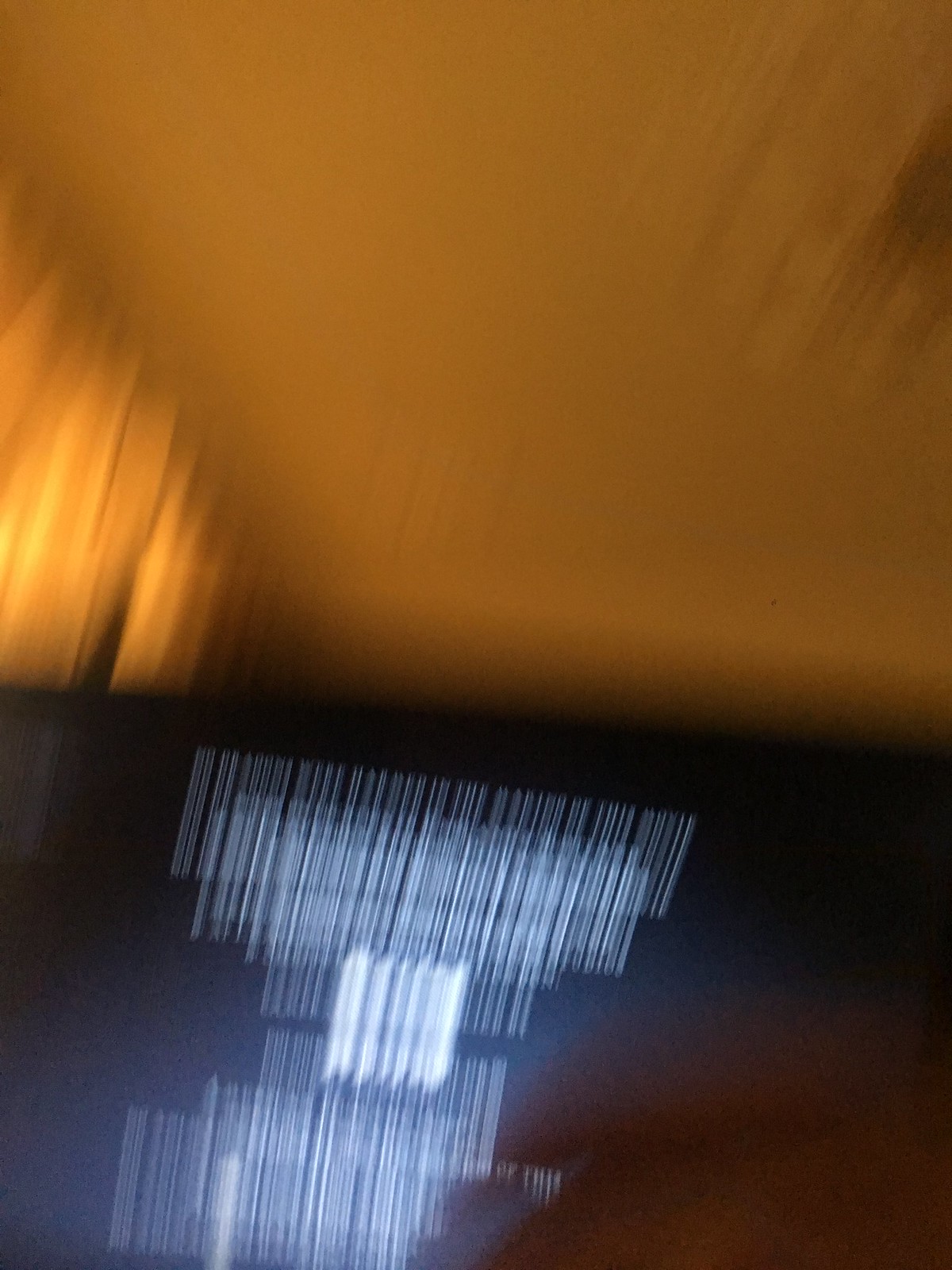The image is an incredibly blurry, underexposed photo with indistinguishable details due to apparent camera motion. The top half of the photo exhibits a dark orange or yellowish-brown color with a darker blur in the top right section. The left upper part appears slightly lighter, possibly illuminated by a light source. The bottom half is predominantly black, except for a dark red area in the bottom right corner. Near this corner, there is a blurry, vertical light source with numerous white lines that transition from thin at the edges to thick and almost solid in the center, forming a shape that resembles a square blur. The overall image lacks identifiable elements, making it hard to discern whether it was taken indoors or outdoors, and what objects or scenes it might represent.